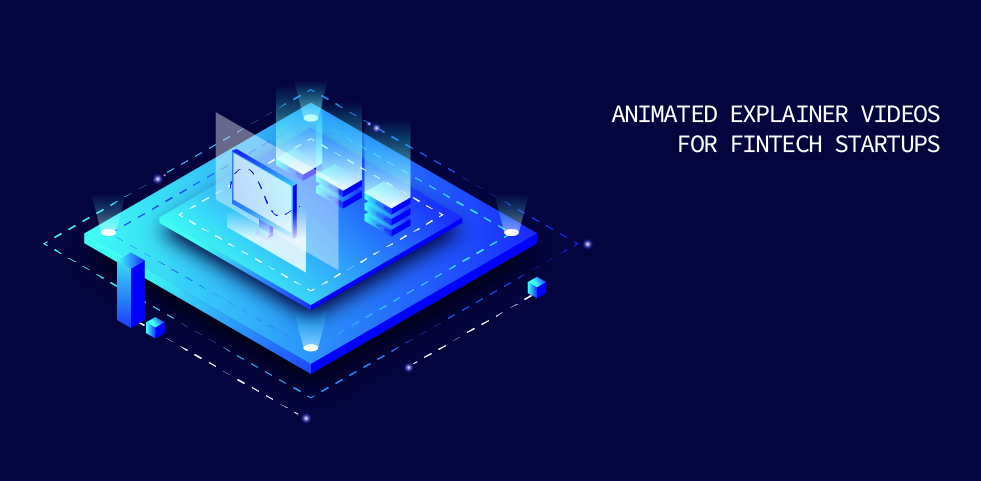The image features a sophisticated graphic design piece set against a dark blue, near-black background, geared towards advertising fintech startup services. Prominently displayed in the upper right-hand corner, in sleek white text, are the words "animated explainer videos for FinTech startups."

The design is centered around two layered blue platforms, creating a striking visual effect. The bottom platform is presented in a stylized diamond pattern, accentuated with hashed lines that trace a square path around it. Each of the platform’s four corners is equipped with a bright spotlight, emphasizing the structure’s contours.

A second, smaller blue platform is stacked atop the first. This upper platform is adorned with three stacks of blocks: a single block, a two-block stack, and a three-block stack, each topped with a tower-like light emitting a luminous glow. Positioned in front of these stacks is an element resembling a computer monitor or screen, complementing the tech-centric theme of the design.

On the left side, various blue squares and hashed lines enhance the visual complexity, adding layers of depth to the overall composition. This meticulously crafted graphic epitomizes a blend of modern aesthetics and functionality, ideal for engaging and educating fintech audiences.